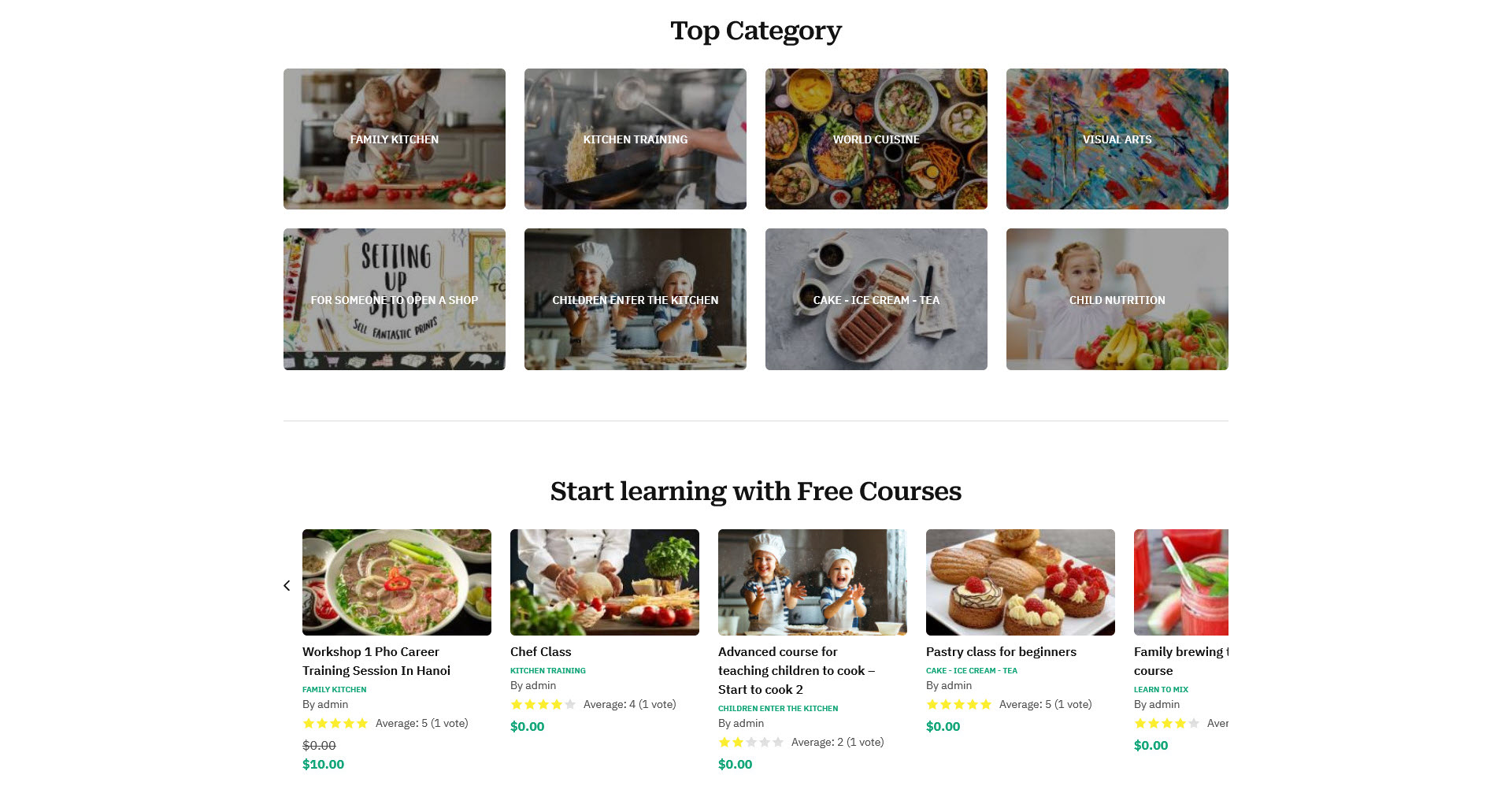In a vibrant family kitchen scene, a woman teaches a young child how to cook. The child, wearing a chef's hat, enthusiastically participates in the kitchen training session. The scene is bustling with various dishes: a person is seen skillfully flipping noodles in a pan, while an array of platters featuring cakes, ice cream, tea, and beautifully arranged fruits and vegetables adorn the countertop.

In the background, a visually striking blue and red painting adds an artistic touch to the room. The setting looks ready for a lively workshop aimed at teaching children the basics of cooking, nutrition, and world cuisine.

A child proudly flexes in front of a nutritious display of fruits and vegetables, highlighting the importance of child nutrition. This setting is part of an introductory, free course designed to inspire young chefs.

Other courses, including a pastry class for beginners and a family brewing course, are available at no cost, showcasing delicious pastries topped with fresh red strawberries and a vibrant red beverage. A chef class features an instructor demonstrating dough handling skills, while a faux career training session details the preparation of a hearty bowl of soup. These classes, led by an admin, have mixed reviews, ranging from two to five stars, emphasizing the community-driven and varied nature of these cooking experiences.

Perfect for anyone looking to start a culinary journey or open a shop, this detailed and dynamic kitchen environment promises education, fun, and delicious outcomes for the whole family.